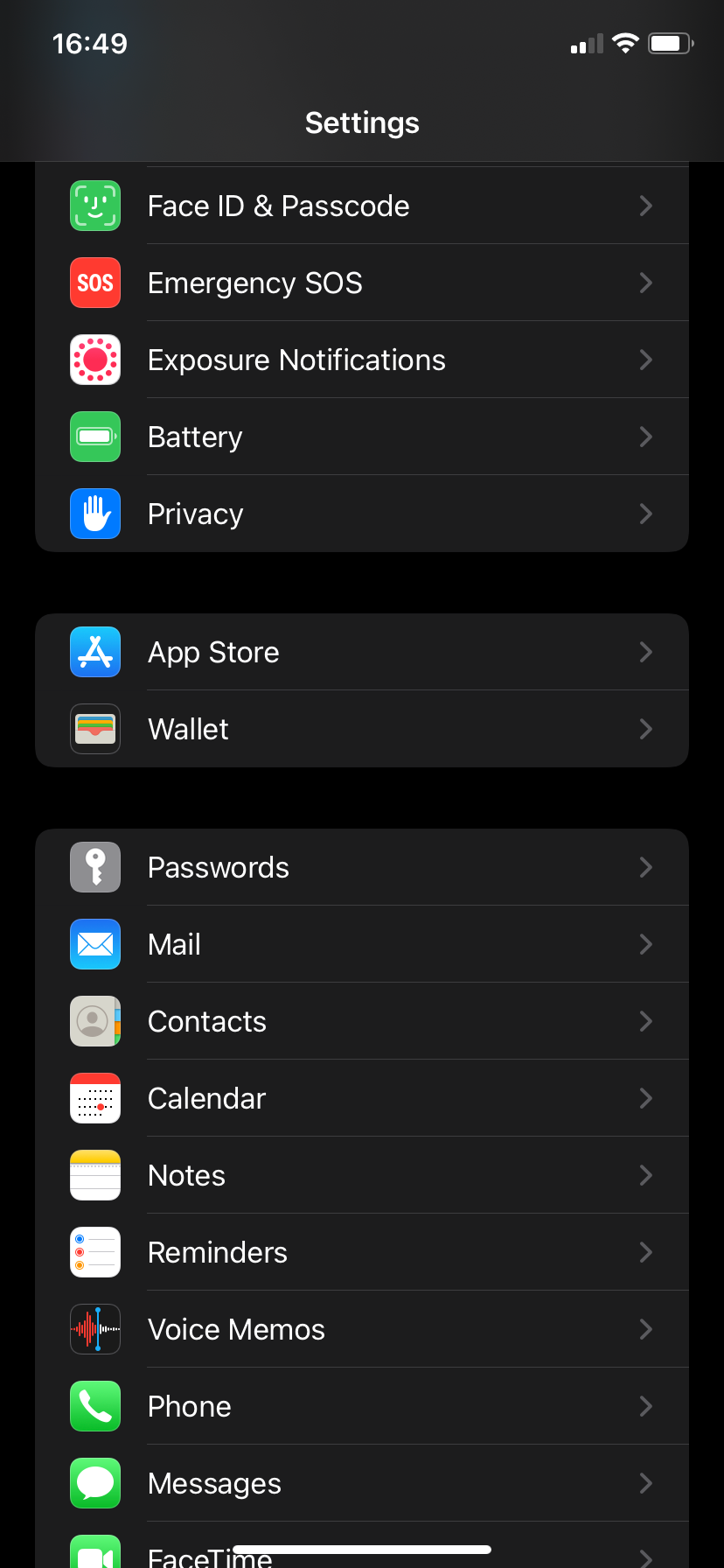The screenshot depicts the settings page of a smartphone with a sleek black background. The top of the screen displays the time as 16:49, with the battery level indicating approximately 80% charge and the signal strength showing two bars. The word "Settings" appears prominently at the top in white, sans-serif font.

Below this heading, a series of rows present various settings options, each accompanied by a corresponding app icon to its left. The list begins with Face ID & Passcode, followed by Emergency SOS, Exposure Notifications, Battery, and Privacy in sequential order. There is a small gap after Privacy, then continues with App Store and Wallet. Another small break leads into the subsequent options: Passwords, Mail, Contacts, Calendar, Notes, Reminders, Voice Memos, Phone, Messages, and FaceTime. Each word in this list is capitalized and consistently formatted in a clean, sans-serif typeface.